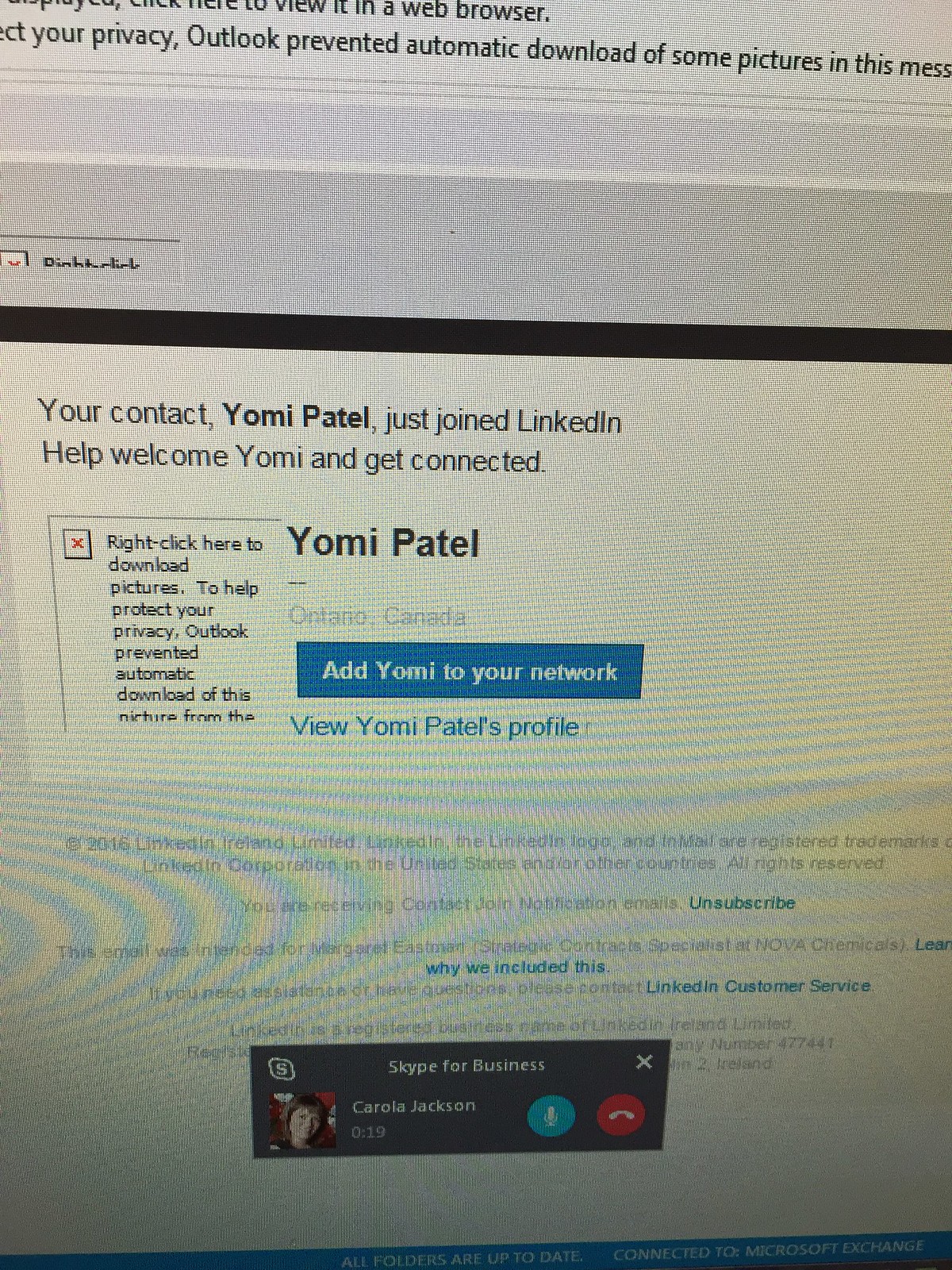This image captures a photograph of a computer screen displaying a LinkedIn notification and other interface elements. The screen appears pixelated, making some details difficult to read. At the top portion of the image, there is a white background with partially visible black text indicating, "Your privacy outlook prevented automatic download of some pictures in this message." Below this, the notification continues with a light gray and a darker gray horizontal bar. Following this, a narrow black line stretches horizontally across the screen.

Central to the image is a LinkedIn notification with clear text that reads: "Your Contact. Yomi Patel just joined LinkedIn. Help welcome Yomi and get connected." Below this, in bold black text, it prominently displays the name "Yomi Patel." There is also a blue rectangle with white text that states, "Add Yomi to Your Network," followed by a blue text link that says, "View Yomi Patel's Profile." Despite the clarity, there are some trademarks and disclaimers below these elements, which are faint and distorted due to the pixelation.

At the very bottom of the image lies a black rectangular box. On the right edge of this rectangle, a white 'X' can be seen in the top-right corner and a white 'S' in the top-left. This box contains text that reads "Skype for Business" along with a name, "Corola Jackson." To the left, there is an image of a woman's face, accompanied by two icons: a blue circle with a microphone and a red circle with a telephone receiver. The black rectangle might also feature lines of white text, which are too small and unclear to discern.